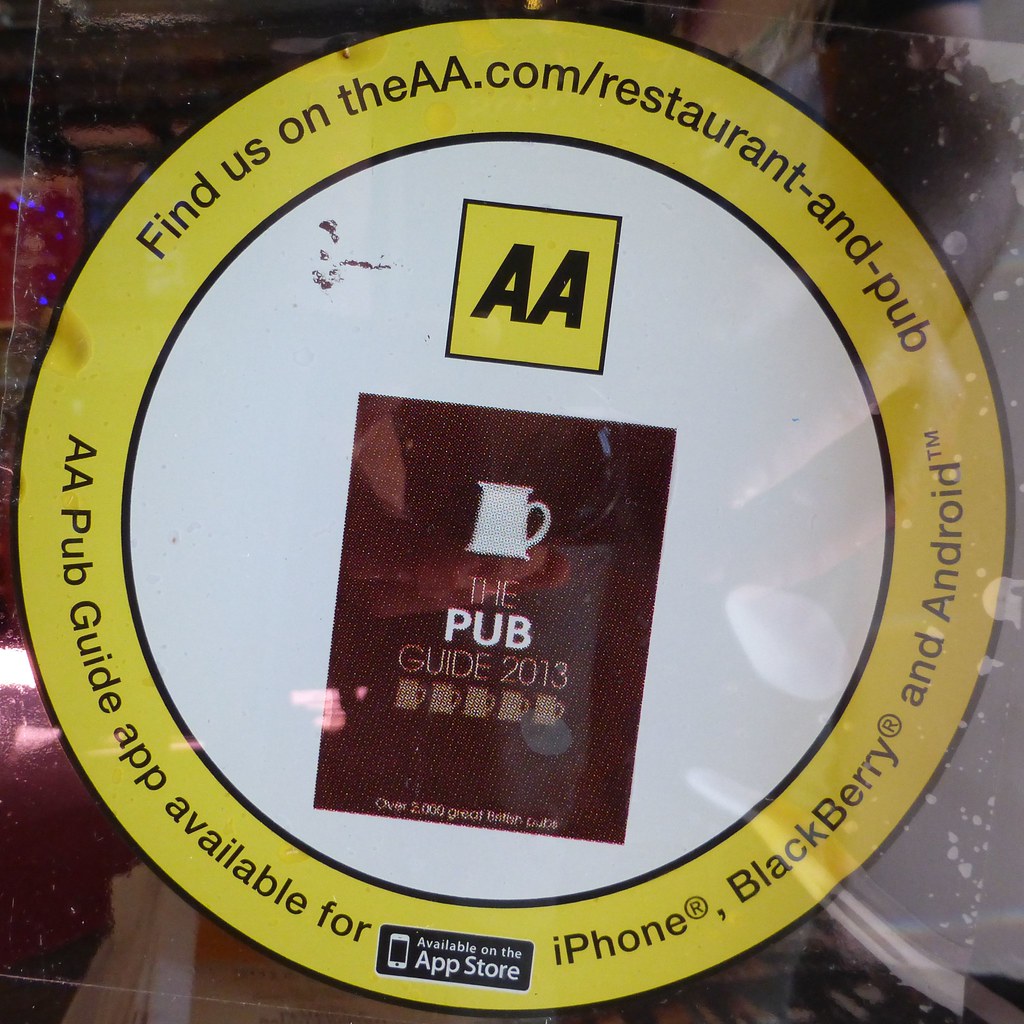The image is a photograph of a circular sticker or sign, likely affixed to a glass window, possibly of a shop or restaurant. The sticker features a yellow outer band and a white central portion. On the yellow band, black text reads: "Find us on AA.com/restaurant and pub," with additional text at the bottom stating, "AA Pub Guide app available for iPhone, Blackberry, and Android." Centrally, within the white portion, there's a smaller yellow square containing the black letters "AA." Directly below, there's a brownish-black square featuring a white coffee mug illustration. Under this mug, white text states, "The Pub Guide 2013," with five smaller coffee mug icons arranged below the text. The sticker's background reveals a blurred interior with some seating arrangements and shelves visible.